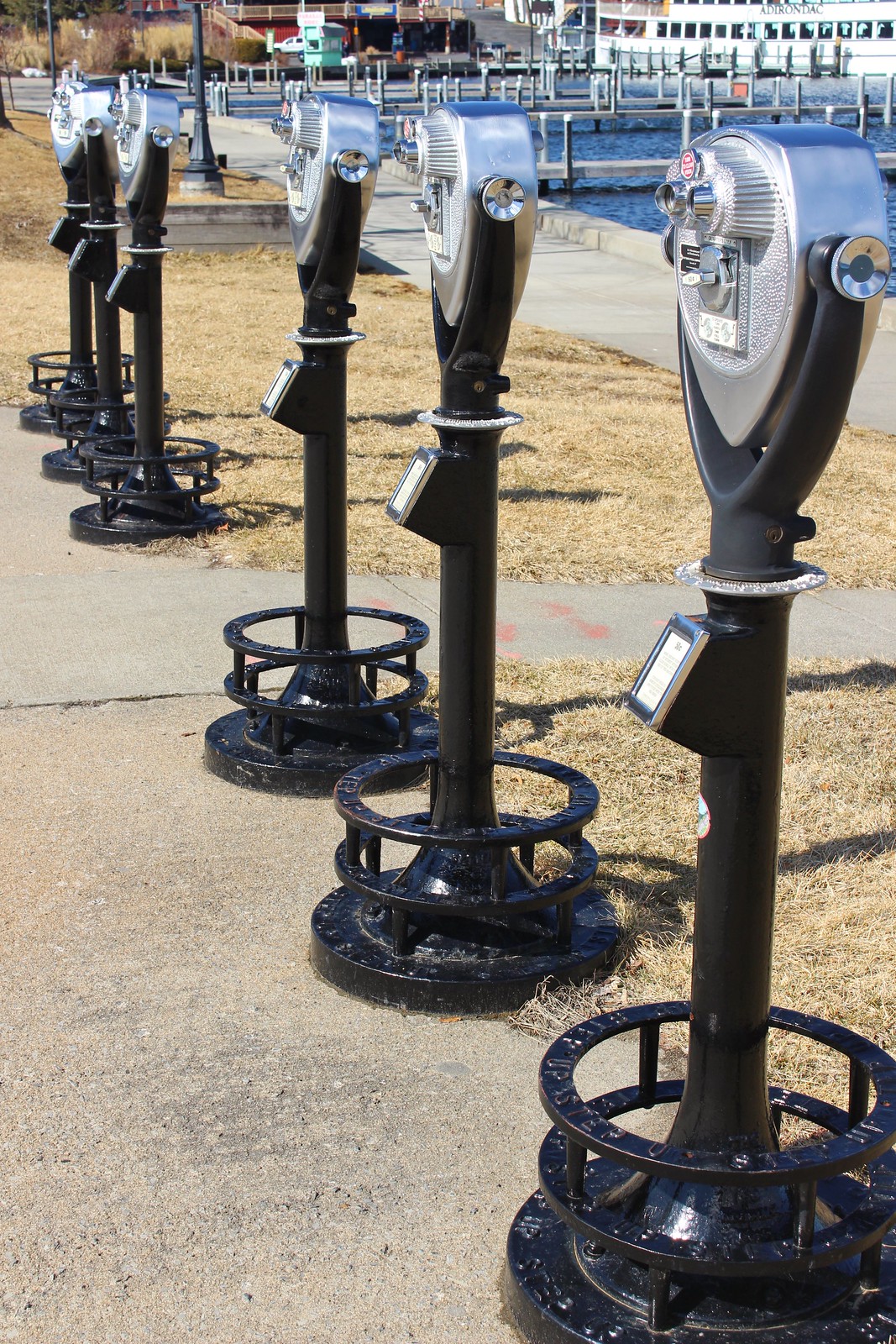This color photograph depicts five large, metallic tourist binoculars, often mistaken for parking meters. Each binocular has a long, black pole stemming from a circular, black base. At the top of the poles, the silver binoculars feature roundish metallic viewing sections with visible dials and slots for inserting coins. The devices are aligned on a sandy-grey cement pathway, which also extends diagonally through the upper left-hand corner of the image. 

Surrounding the pathway, there is dried, browned-out grass, suggesting a late fall or early winter setting. Behind the binoculars, a blue waterway, possibly a canal or river, comes into view along with indications of docks or a marina — including a distant boat. The water displays slight rippling effects. Additionally, a metallic structure, likely a fence or bridge, with vertical and horizontal lines can be seen in the upper left corner of the image. The background features various buildings bordering the water, enhancing the scenic viewing experience that the binoculars offer.